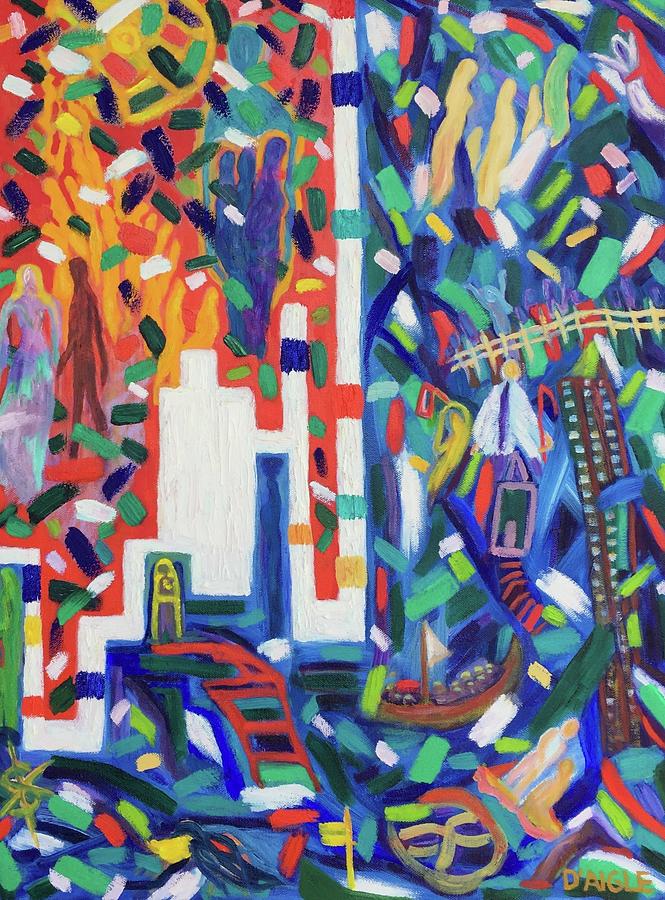This vibrant and bustling abstract painting, potentially created using acrylic or oil pastels, features an intense, colorful composition with predominantly warm orange tones in the upper left corner and cool blue hues on the lower right. The chaotic background is speckled with bright strokes of white, blue, green, yellow, red, and pink, creating a visually striking, crowded image. The backdrop transitions from red along the top left to a backwards L-shaped swath of blue covering the right and bottom left sections.

Among the abstract smudges and lines are indistinct objects and faintly recognizable silhouettes. On the left, one can discern the outline of a woman in a white dress with blonde hair and a brown silhouette of another figure. To the right, another silhouette appears to represent a person wearing a shirt and tie, seemingly occupied with a drawing. The painting also features a hand-like figure at the bottom right corner where the letters "D'AIGLE" are inscribed. Additional details include a central white line extending towards the left, surrounded by a scatter of black and white speckles, humorously described as "salt and pepper." In the background, amid the vibrant hues, there also seem to be abstract representations of buildings and celebratory confetti-like sprinkles.